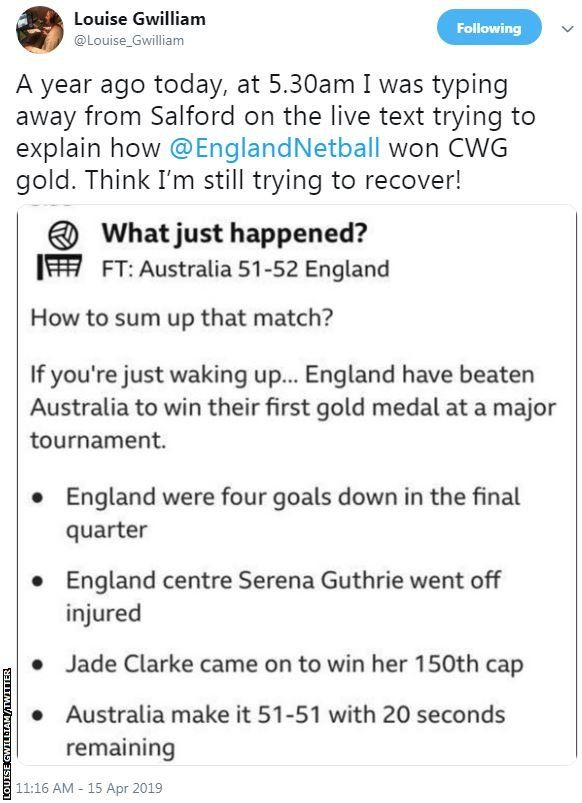In the upper left corner, there is a profile picture depicting a person sitting in front of a computer, wearing headphones. To the right of the profile picture, the name "Louise G. William" is displayed followed by the username "@LouiseGWilliam" and a blue circle indicating "Following."

The message reads: 
"A year ago today at 5:30 a.m., I was typing away from Salford on live text, trying to explain how @EnglandNetball won the CWG gold medal. I think I'm still trying to recover!"

To the left of this message, there is an image showing a ball going into a net. Beside this image, a caption says, "What just happened? FT: Australia 51 - 52 England."

Below this, another caption reads:
"How to sum up that match? If you're just waking up... England have beaten Australia to win their first gold medal at a major tournament."

Further details are provided in the form of three circular icons:

1. A black circle to the left, with text to the right explaining, "England were four goals down in the final quarter."
2. Another circle noting, "Then England centre Serena Guthrie went off injured."
3. The final circle states, "Jade Clarke came on to win her 150th cap." 

Concluding with, "Australia made it 51 - 51 with 20 seconds remaining."